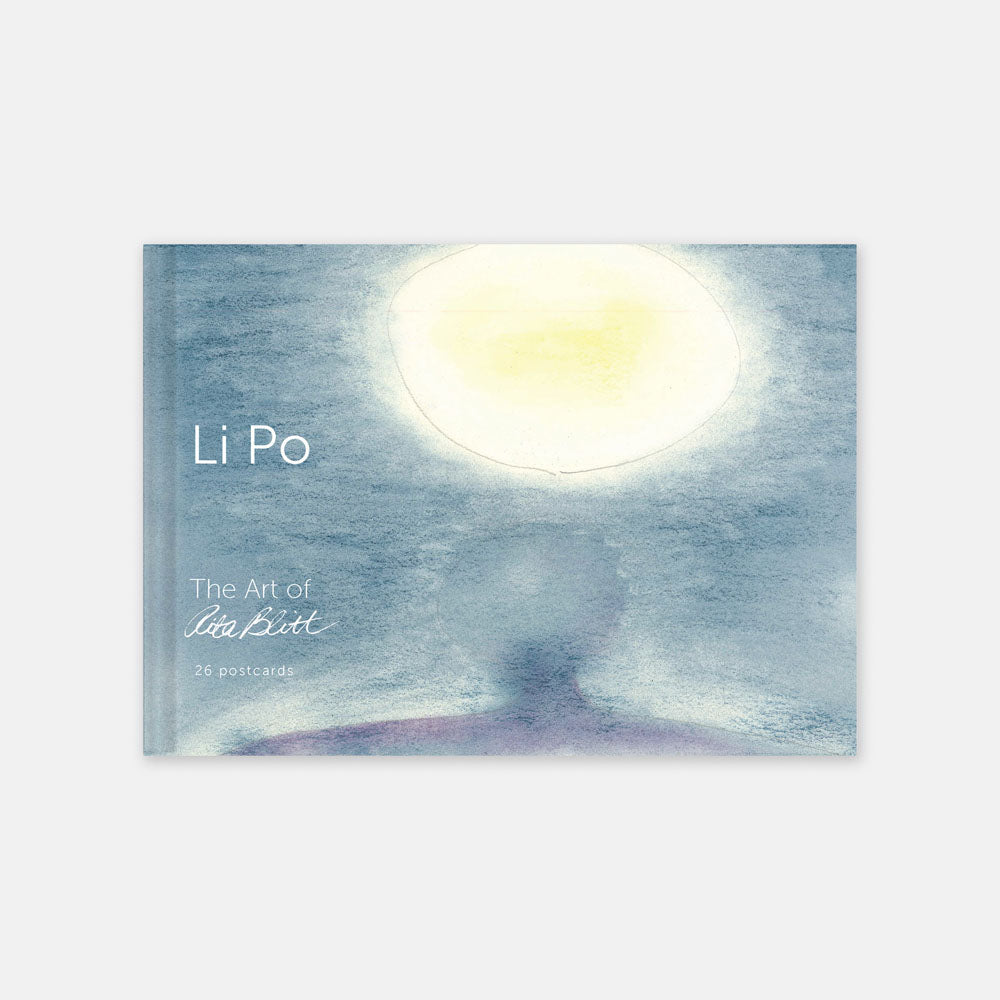The image depicts the cover of a book titled "Li Po: The Art of Ada Blit." The title "Li Po" is prominently displayed on the left side of the cover, with "The Art of Ada Blit" written below it in a cursive, signature-like font. Additionally, it mentions that the book contains "26 postcards."

The cover itself features a striking piece of art. The background is a gradient of blue, representing a serene sky, blending into a purplish hue in the lower half. This section appears somewhat abstract, resembling either the silhouette of the back of a person's head and shoulders or a stylized rounded hill. Above this is a large, lemon-shaped orb that is yellowish in color, emitting a soft glow that extends beyond its outline, reminiscent of a sun or moon.

Overall, the cover art combines elements that evoke both a celestial and terrestrial feel, making it both visually engaging and artistically unique.